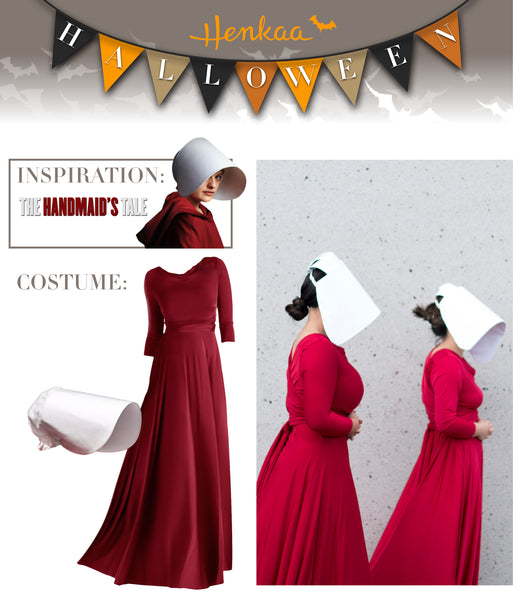The image showcases a detailed display for a Halloween costume inspired by "The Handmaid's Tale." At the top, an orange banner reads "Henka Halloween," featuring a series of upside-down triangle pennants that spell out "HALLOWEEN." The triangles alternate in a festive pattern of black, orange, tan, black, orange, and a different shade of orange, embodying traditional Halloween colors.

Below the banner, the costume itself is presented through multiple views. The central element is a red dress complemented by a white bonnet-like hat that obscures the wearer's face, creating an authentic "Handmaid's Tale" look. The display includes several images: one showing just the dress, two of different women wearing the costume, and an upper image focusing on a face covered by the bonnet. The word "Costume" is prominently featured on the left side of the display, highlighting the garment's purpose for Halloween festivities.